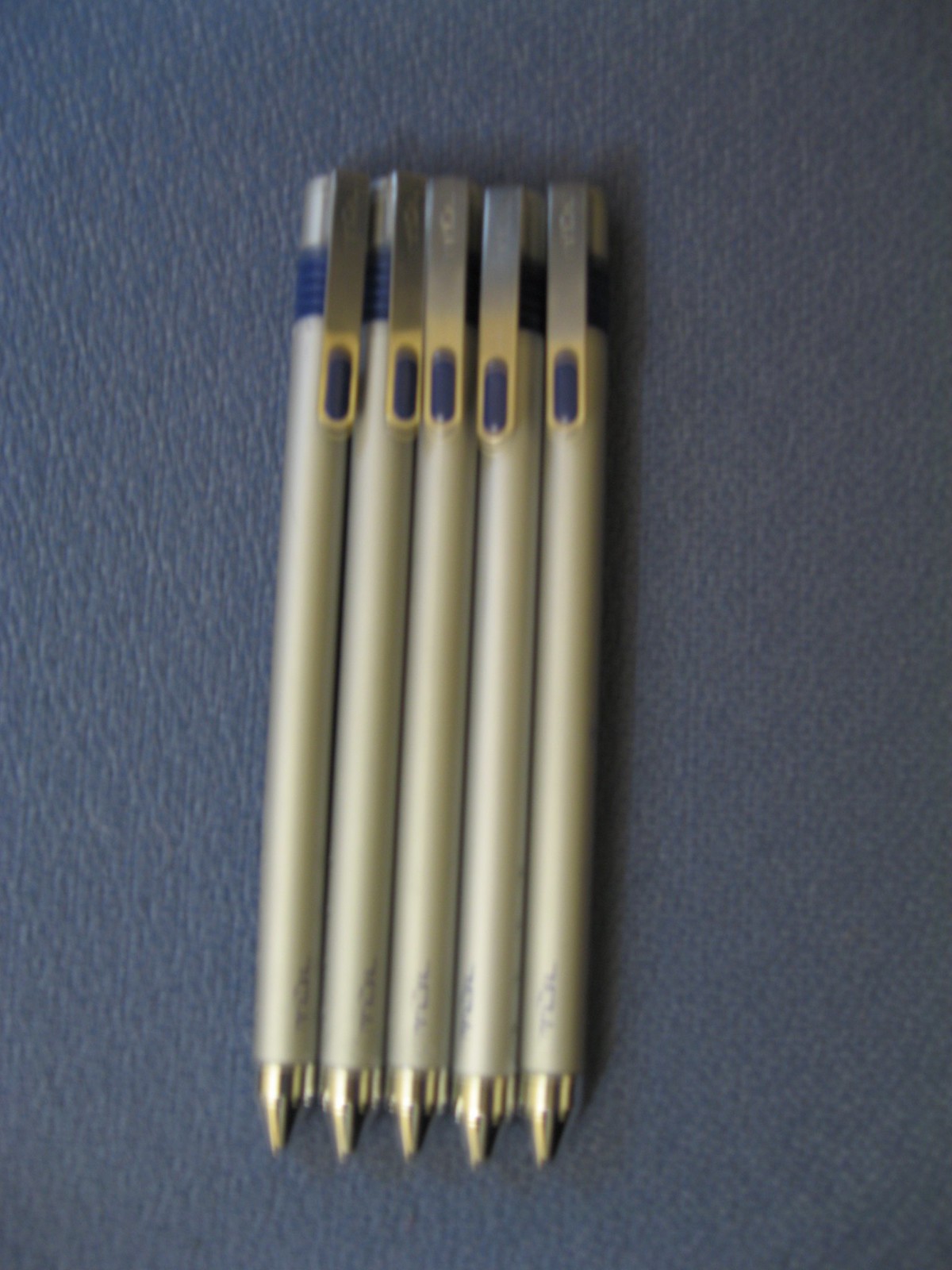The image depicts five retracted ink pens arranged vertically side-by-side on a blue textured background. Each pen features a sleek silver body with a shiny silver tip and a small strip of thin blue text towards the bottom. Near the upper section, the pens have a textured blue band wrapping around them. This is accompanied by a metal pocket clip, which incorporates a blue strip at its base and a small amount of white text at the top. The pens also have a distinctive blue button near the top end. The overall appearance suggests that these pens may be promotional items.